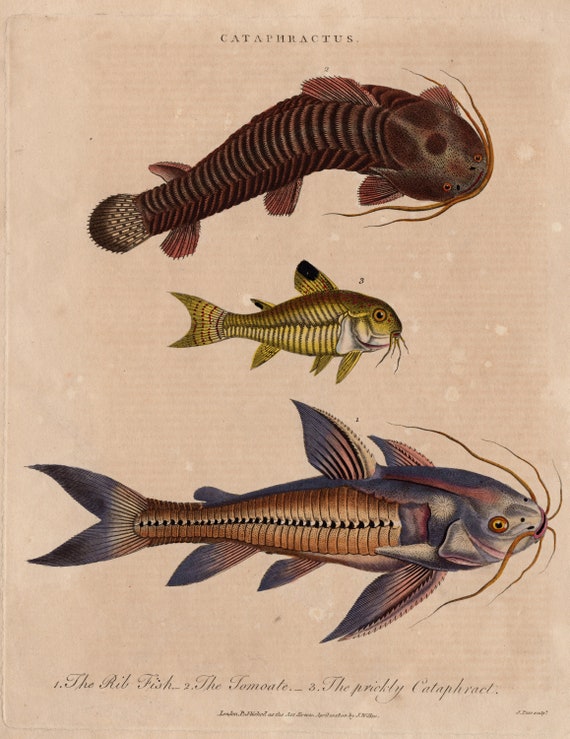This vintage-style color illustration, presented in portrait orientation, showcases three distinct catfish of varying sizes and peculiar designs, all centered one over the other. Across the top, in small black letters, is the technical term 'Cataphractus.' The background features a dark cream color with an aged, spotted texture adding to its antique appeal.

At the top of this illustration is a brown catfish with a very sloped nose and dull orange stripes running down its back. It has long brown whiskers and spans three-quarters of the width of the image, with its face pointing to the right and its tail to the left.

The middle catfish is much smaller and gold-colored, bearing black stripes on its back. This fish also presents in profile with whiskers on the front, its nose pointing right and tail left.

At the bottom is the largest catfish with a silhouette that extends almost the full width of the image. This fish is adorned with a beige body covered in vertical scales, colorful fins along the top and bottom, and whiskers so long they stretch nearly to the right edge of the illustration. Across the bottom of the image is a script description detailing the fish types.